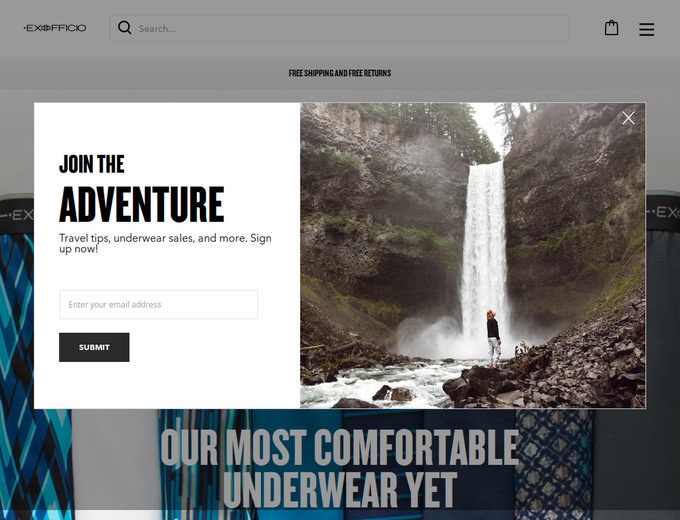A screenshot from the ExOfficio website showcases various elements of the online storefront. In the top left corner, the ExOfficio logo is prominently displayed beside a search bar. Moving to the right, a shopping bag icon and a menu icon consisting of three horizontal black lines are visible. Just below this header, a horizontal gray banner spans the page, announcing "Free Shipping and Free Returns" in clear, bold text.

A pop-up box occupies the center of the screen, inviting visitors to "Join the Adventure" for access to travel tips, underwear sales, and more. The pop-up includes a field to enter an email address and a prominent black "Submit" button for easy subscription.

Dominating the background is an evocative image of a woman standing at the base of a waterfall, gazing upward at the cascading water descending over rugged rocks. This scenic backdrop enhances the site's inviting and adventurous aesthetic. Below the image, a tagline reads, "Our Most Comfortable Underwear Yet," emphasizing the website's product focus.